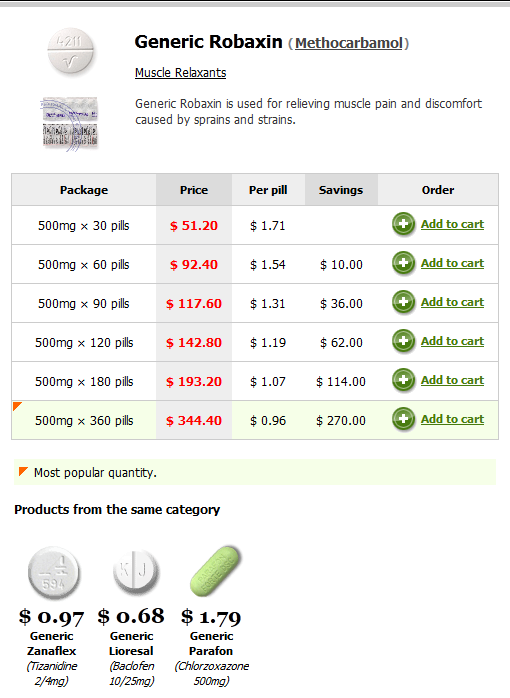This is a photo of a website comparing drug prices, presented in a portrait orientation. The image does not have borders along the left, right, or bottom edges, but it features a gray horizontal border along the top with a thin black line above it. 

Below this border, there's a white section displaying an off-white circular pill with the imprint "4211" above a dividing line and a stylized "V" underneath it. To the right of the pill image, the text reads "Generic Robaxin (Methocarbamol)" followed by the category "Muscle Relaxants." Beneath this information is an image resembling a stamp that states: "Generic Robaxin is used for relieving muscle pain and discomfort caused by strains and sprains."

Further down, there's a grid with gray header boxes labeled "Package," "Price," "Per Pill," "Savings," and "Order." The grid lists the dosage, consistently 500 milligrams, alongside the number of pills in each package. It also displays the combined price, the price per pill, and the potential savings for each package option. The "Order" column features a green circle with a white plus sign labeled "Add to Cart" for each package. 

The bottom package option, 360 pills at 500 milligrams each, is highlighted in green, indicating it is the most popular choice as noted at the bottom of the grid.